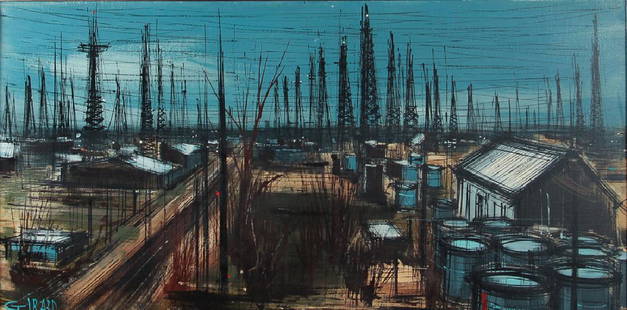The image is a colorful drawing, likely created with colored pencils. It depicts an industrial scene set against a deep blue, nighttime sky, speckled with patches of white clouds. Dominating the background are numerous black steel girder towers, possibly oil derricks or ship masts, numbering around 20 to 25. These towers create a dense, structured skyline.

In the foreground, a wooden dock stretches across the image, with various buildings and tents set up along it. Particularly noticeable on the right side is a small, white metal shack surrounded by blue barrels or drums, with around eight or nine drums clustered both in front and behind the structure. A road runs down the left side of the scene, flanked by additional buildings. The overall atmosphere of the drawing is shadowy and muted, underlining the nighttime setting of this bustling dockside or industrial area.